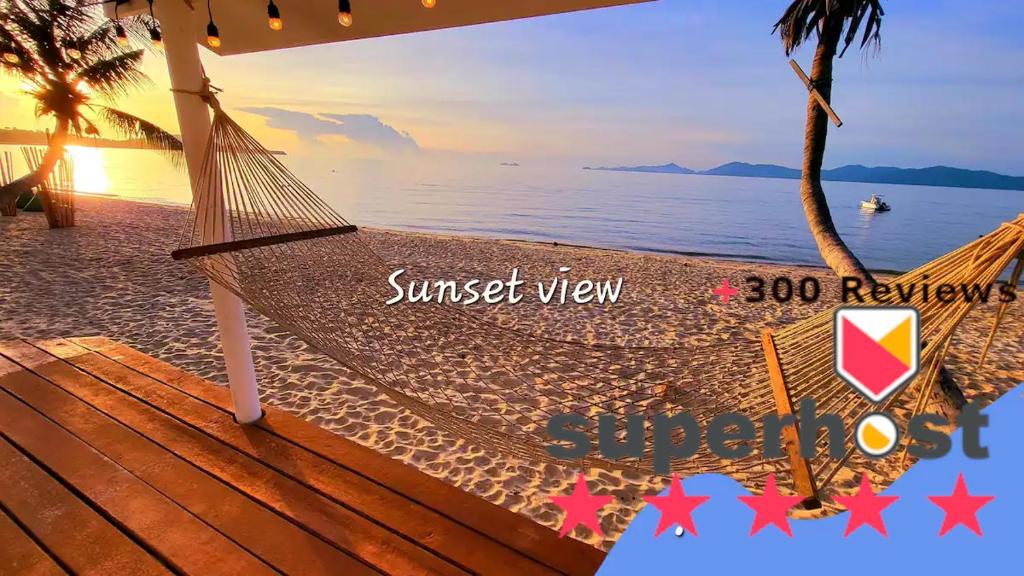This captivating outdoor photograph serves as an advertisement highlighting a serene coastal retreat. Dominating the lower left-hand corner is a weathered redwood deck adorned with an inviting, empty hammock, suspended securely between sturdy wooden posts. Overhead, a series of delicate lights dangle along the edge of an open roof, adding a touch of twinkle to the ambiance.

Stretching out from the deck is a picturesque sandy beach leading to an expanse of almost calm, beautiful water. In the background, a lone boat languidly floats just off-center, enveloped by the tranquil ocean waves. A magnificent panorama unfolds beyond the water, showcased by majestic hills and mountains under a vibrant blue sky. 

Prominent on either side of the frame are two palm trees; one leans gracefully, while the other stands directly in front of the radiant sun, either setting or rising, casting a golden glow across the scene. Superimposed on the photograph is the phrase "Sunset View" in elegant white text. To the right, a graphic proudly announces "300 reviews," and at the bottom, the words "Superhost" are displayed alongside an impressive five-star rating and a distinctive award badge. The badge, resembling an inverted shield with a diagonal red and yellow stripe and an exclamation mark where the "O" is a combination of half yellow, half white, signifies the premium status of the host. This meticulous composition exudes a sense of tranquil luxury, inviting viewers to indulge in the breathtaking sunset view and unparalleled hospitality.